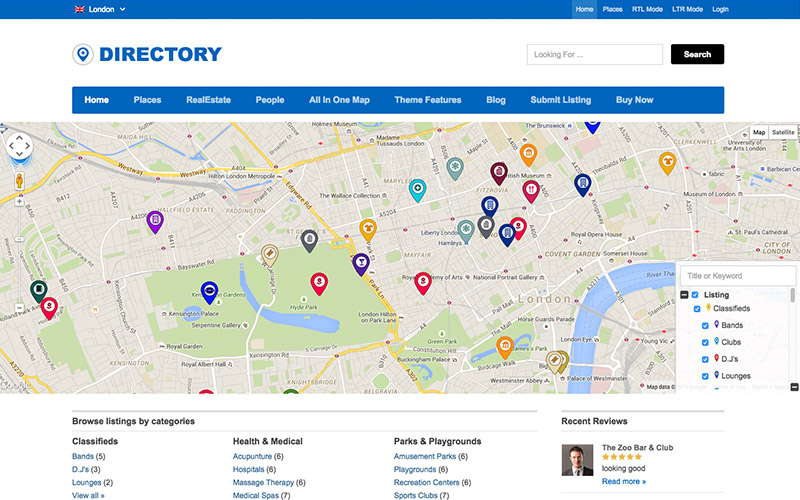This screenshot depicts an interactive property search map interface, likely focused on the London area. At the top of the page, there's a thin, full-width blue navigation bar. On the left side of this bar, there's a Union Jack icon followed by the word "London" and a dropdown arrow, suggesting a feature to select different cities or areas. To the right, menu options include "Home," "Places," "RTL mode," "LTR mode," and "Login," with "Home" currently highlighted.

Below this primary navigation bar, there's another blue bar, though it's not full-width. This secondary menu includes options such as "Home," "Places," "Real Estate People," "All in One Map," "Theme Features," "Blogs," "Submit Listing," and "Buy Now." 

Beneath these menus, there's a directory pane on the left with a map icon, and to its right, a search bar labeled "Looking For," accompanied by a black "Search" button. The central content of the page is dominated by a map populated with various icons in different colors: blue and red. These icons represent different categories indicated by symbols such as dollar signs, houses, tickets, and food, although the legend for these icons is not visible.

The map is clearly centered on London, showcasing notable landmarks such as Hyde Park and the River Thames. 

On the lower right of the map, a section labeled "Searching for Listings" offers categories like classifieds, bands, clubs, DJs, and lounges, though no specific filters appear to be selected.

Further down, below the map, is a section titled "Browse Listed by Categories," featuring options like "Classifieds," "Health and Medical," and "Parks and Playgrounds," with the number of results available listed in blue text.

To the far right, there's a "Recent Reviews" panel displaying reviews of different locations. One such review features a man and highlights the "Zoo Bar and Club," which has received a five-star rating along with a brief comment, "looking good," and a "Read More" option.